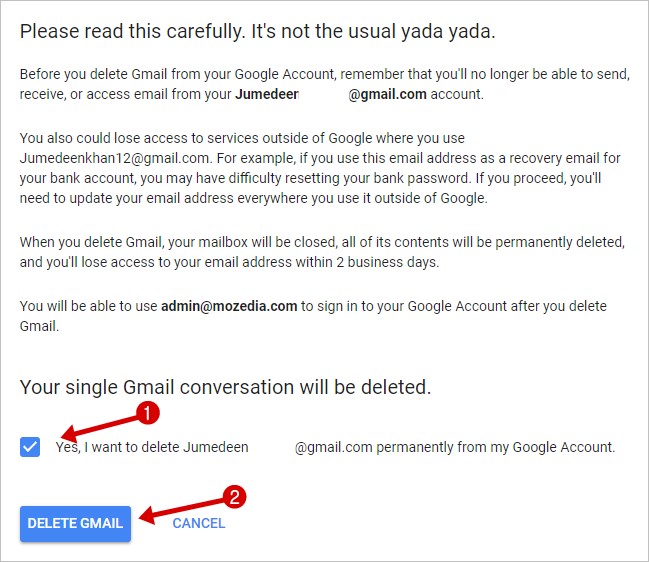Before deleting your Gmail account, it is crucial to understand the ramifications. Deleting your Gmail account means you will no longer be able to send, receive, or access emails from your "junedean@gmail.com" account. Additionally, you may lose access to non-Google services where this email is used, such as for bank account recovery. It's important to update your email address in all places where you use it outside of Google before proceeding. 

Once you delete your Gmail, your mailbox and all its contents will be permanently deleted, and you will lose access to your email address within two business days. However, you will be able to use "admin@mozilla.com" to sign into your Google account after the deletion.

The image has a red arrow labeled "1" pointing to a blue checkbox, and a red arrow labeled "2" pointing to the "Delete Gmail" button. The text is written in black, outlining the steps and implications of deleting the Gmail account.

Yes, I want to permanently delete "junedean@gmail.com" from my Google account.
[Delete Gmail] [Cancel]